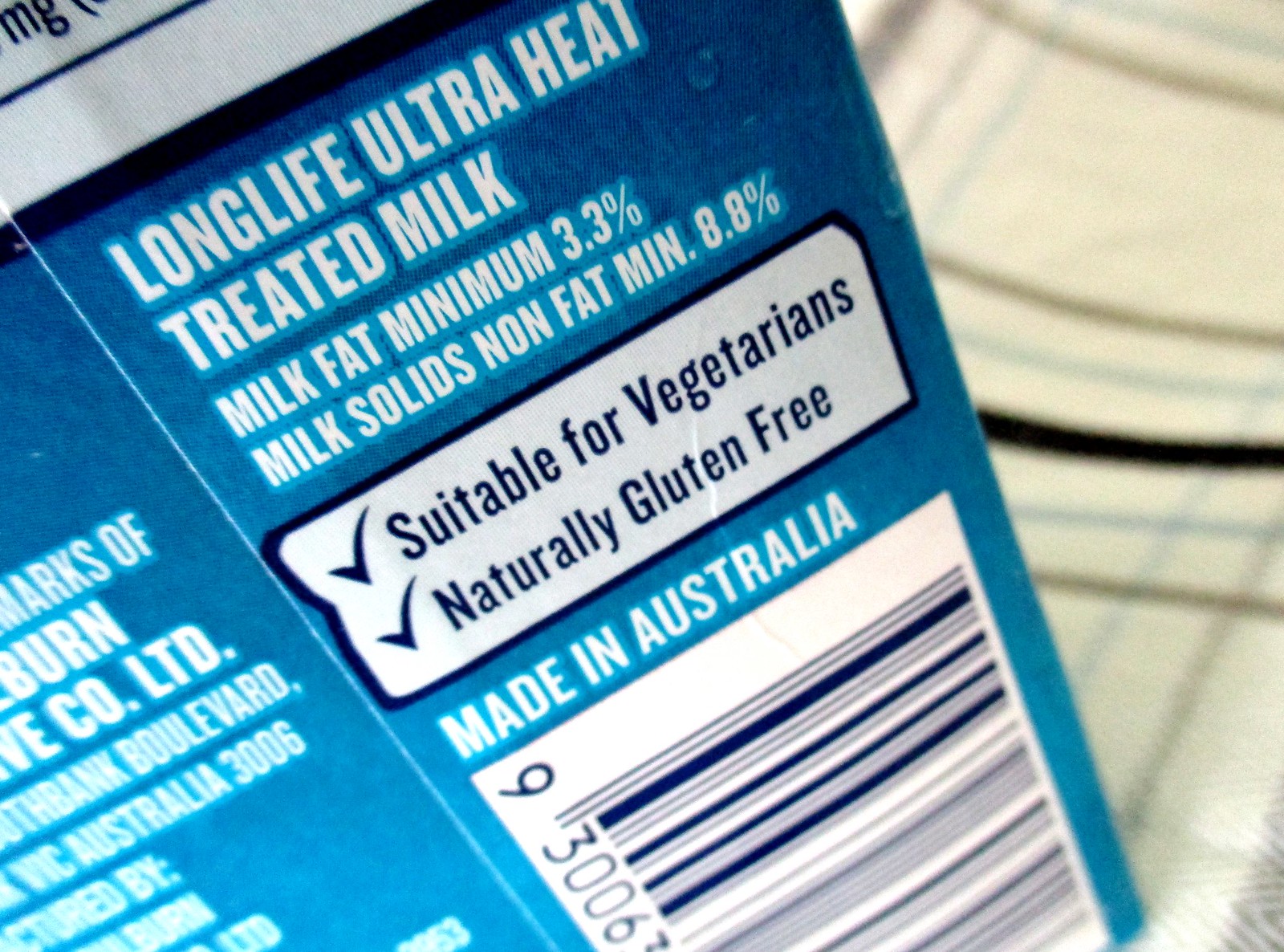This detailed close-up image showcases the back of a blue and white carton of Long Life Ultra Heat Treated Milk. At the top of the carton, the text reads "Long Life" and "Ultra Heat Treated Milk." The carton clearly states "Milk fat minimum 3.3%" and "Milk solids nonfat minimum 8.8%." Prominent on the packaging is a white rectangular section with rounded edges that features two check marks: one indicating the product is "Suitable for Vegetarians" and the other confirming it is "Naturally Gluten Free." Additionally, the text "Made in Australia" is prominently displayed within a white box with a blue border. There's a blue and white barcode visible on the carton as well. Along the left side of the carton, there is more information about the manufacturer, including partial text about "Burn Co Limited, Alth Bank Boulevard, Vic Australia 3006," suggesting the product's origins and distribution details. The carton rests on a fabric that resembles a bedsheet or tablecloth with a white background featuring gray, light blue, and thick black stripes.